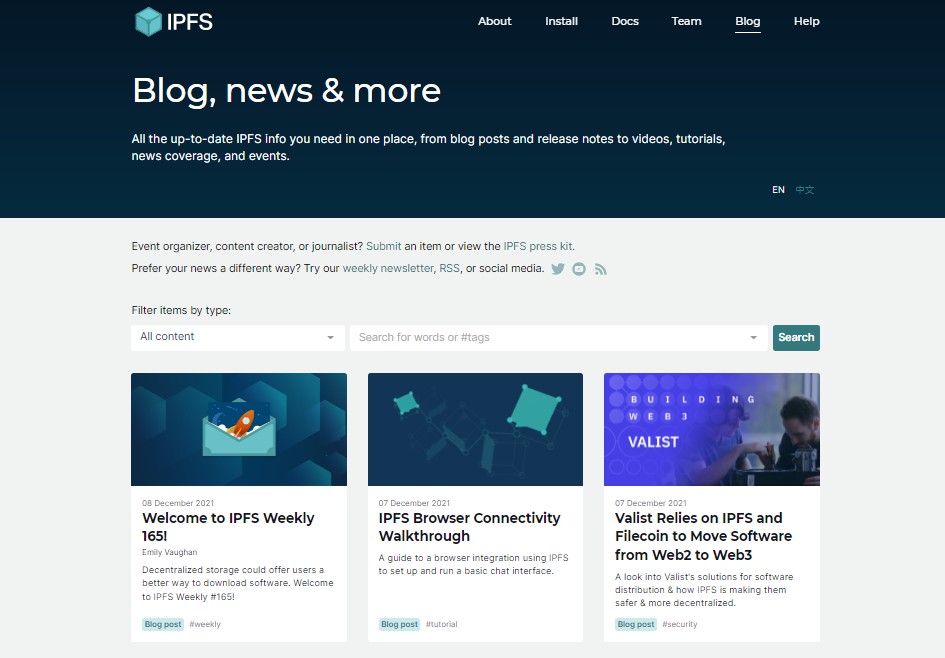This screenshot captures a segment of a website with a dark blue header and white text. The header features a blue cube logo with "IFFS" in the top left corner. Adjacent to the logo, navigation options are listed: About, Install, Docs, Team, Blog (underlined), and Help. Below this, in a larger white font, it reads: "Blog", "News", and "More", promoting the latest IFPS information. The section explains that visitors can find various content, including blog posts, release notes, videos, tutorials, news coverage, and events, all available in English.

The main body of the page has a grey background with black text catering specifically to event organizers, content creators, and journalists. The text invites users to submit items or view the IFPS price list, and offers a press kit. It also provides information on alternative ways to consume news, such as a weekly newsletter, RSS feeds, or social media, with corresponding buttons for social media platforms.

A search section follows, allowing users to filter content by type, search for specific words or tags using hashtags, and initiate the search with a dark green and white search button on the right.

Three blue rectangles are displayed prominently. The left rectangle contains an envelope with an image resembling a bird, labeled "Welcome to IFFS Weekly 1651", though the accompanying text is too small to read. The central rectangle features two light turquoise pillows against a blue background, titled "IFFS Browser Connectivity Walkthrough," again with unreadable smaller text underneath. The right rectangle depicts a whitelist with small blue and white icons, suggesting collaborative work. The text below describes that the whitelist utilizes IPFS and Filecoin technologies to transition software from Web2 to Web3.